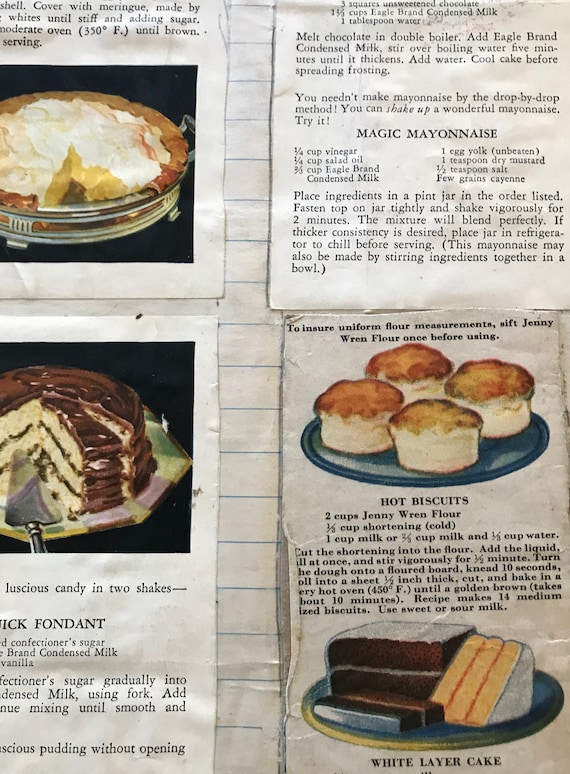The image is a collage of four distinct recipe pages, likely cut from an older printed cookbook, arranged against a background of lined paper. The recipes are detailed and each is accompanied by either a photograph or an illustration of the finished dish. 

In the upper left quadrant, there is a recipe for a Bavarian cream pie featuring a lemon meringue pie photo. Below it, positioned in the lower left quadrant, is a photograph of a three-layer chocolate frosted cake with a corresponding recipe for a quick fondant that involves mixing confectioner's sugar and condensed milk until smooth.

The right side of the collage holds two more recipes. The upper right quadrant displays the recipe text for 'Magic Mayonnaise,' which consists of ingredients such as vinegar, salad oil, and an unbeaten egg yolk, with detailed instructions to shake the mixture vigorously. Below this, in the lower right quadrant, are recipes for 'Hot Biscuits' and 'White Layer Cake.' This section includes an illustration of hot biscuits and a photograph of a white layer cake, accompanied by their respective recipes.

Overall, the collage captures a nostalgic collection of vintage recipes for various baked goods and condiments, pieced together in a visually appealing and detailed montage.